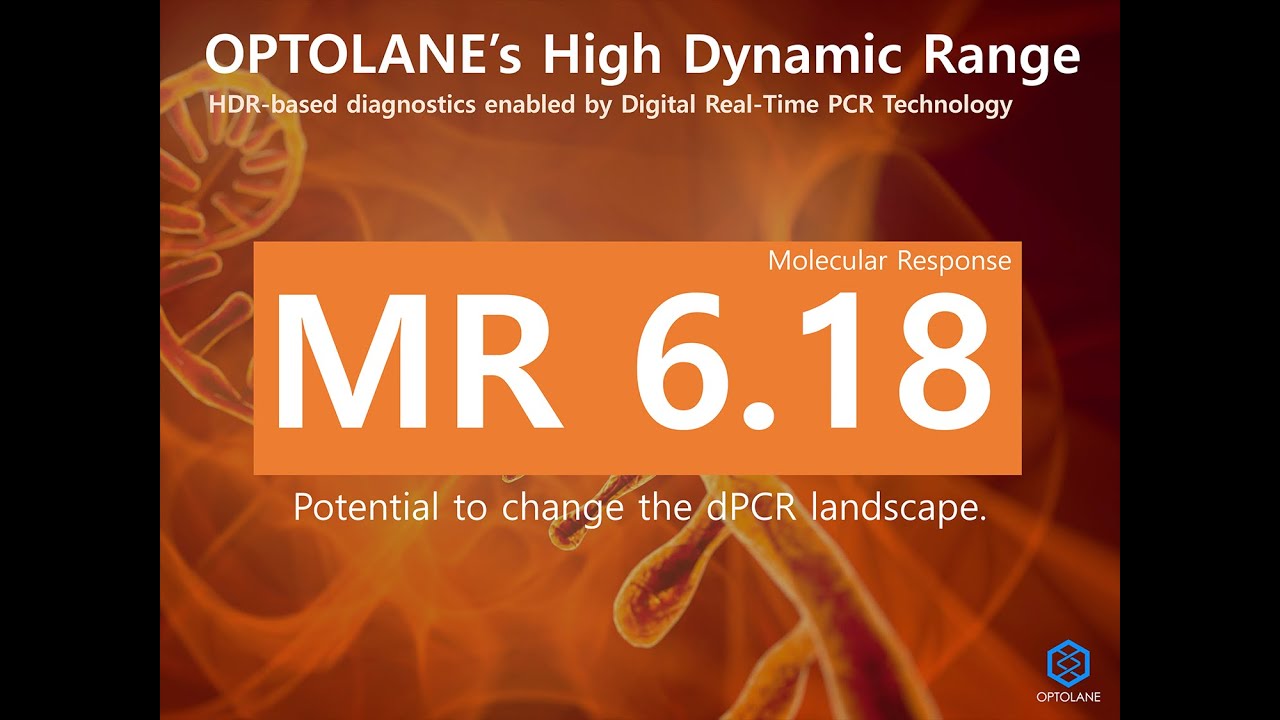The image appears to be a detailed promotional slide or web page screenshot for an advanced diagnostic tool. The background features a striking orange color scheme with what seems to be a microscopic or digitally created image of a DNA strand. Prominently displayed at the top in white text is “OptaLane’s High Dynamic Range,” followed by “HDR-based diagnostics enabled by digital real-time PCR technology.” At the center of the slide, within an orange rectangle, the text reads “MR6.18” with “molecular response” above it, and below it, in white text, it states “potential to change the dPCR landscape.” In the bottom right corner, there is a small blue insignia with the brand name “OptaLane.” This comprehensive presentation suggests the slide is advertising a high-strength microscopy tool, aimed at revolutionizing the field of digital PCR diagnostics through sophisticated molecular response technology.